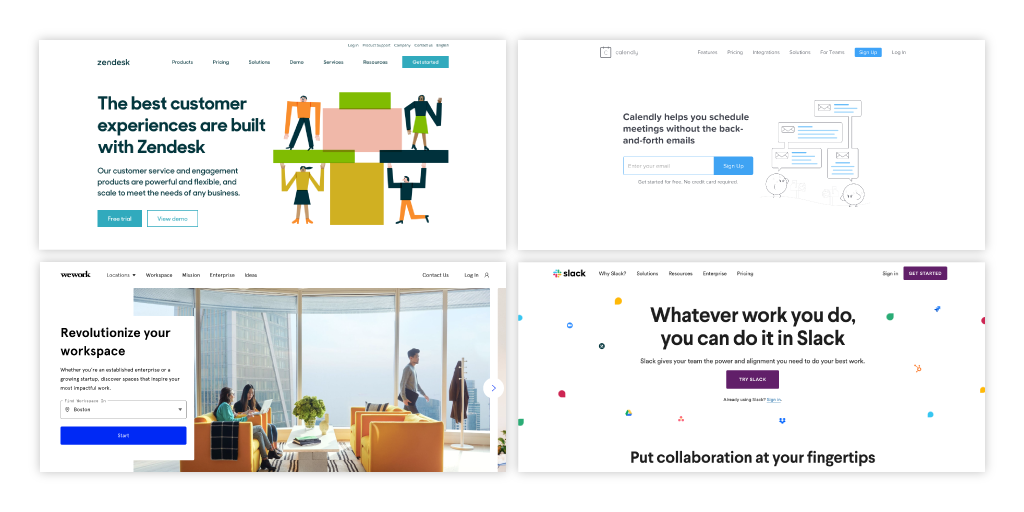The image is divided into four quadrants showcasing different software tools that enhance work productivity. 

In the upper left-hand quadrant, Zendesk is highlighted with a green and yellow color scheme. The tagline reads, "Zendesk: The best customer experiences are built with Zendesk. Our customer service and engagement products are powerful and flexible, scaling to meet the needs of any business."

The upper right-hand quadrant features Calendly, emphasizing its user-friendly scheduling capabilities. The caption states, "Calendly helps you schedule meetings without back-and-forth emails. Sign up to streamline your scheduling process."

In the lower right-hand quadrant, Slack is showcased. The caption reads, "Slack: Whatever work you do, you can do it in Slack. Slack gives your team the power and alignment needed to do your best work. Put collaboration at your fingertips with the 'Try Slack' button in purple."

Lastly, the lower left-hand quadrant highlights WeWork. The caption encourages, "WeWork: Revolutionize your workspace. Whether you’re an established entrepreneur or a growing startup, find spaces that inspire your most productive work."

Each quadrant effectively communicates the unique value proposition of these popular work-oriented applications.